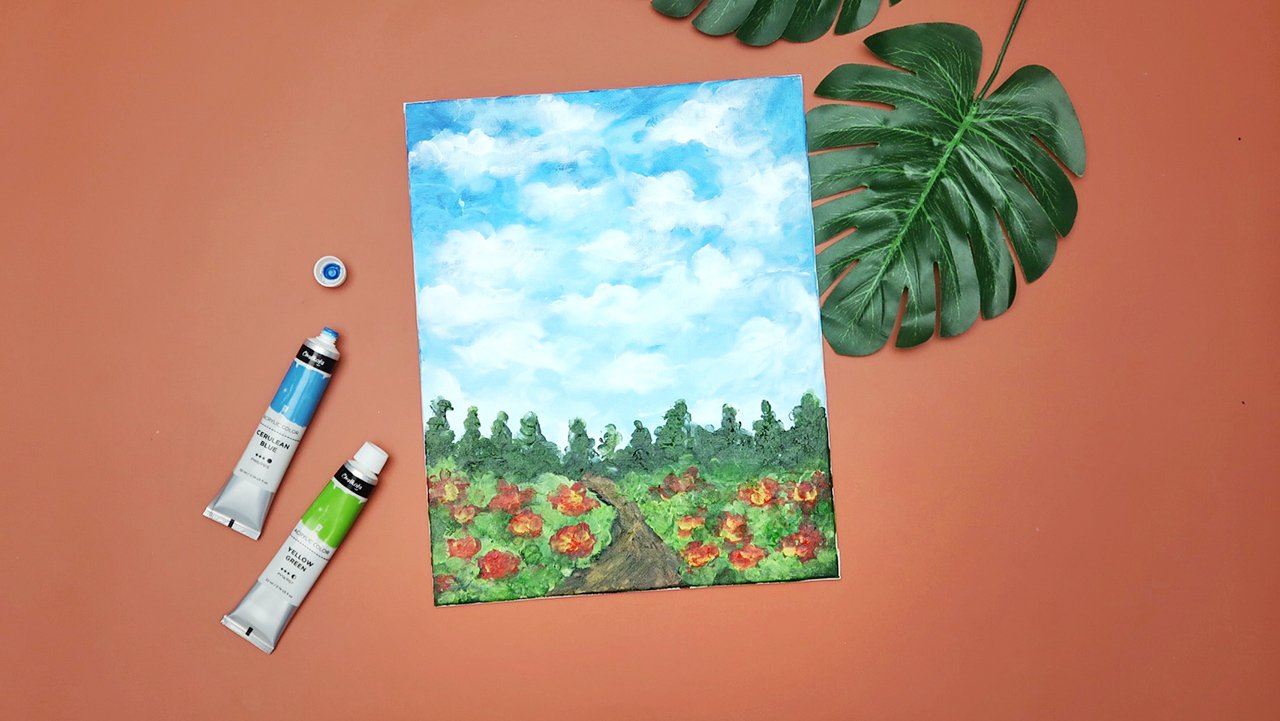This image is a top-down photograph of a small, amateurish landscape painting on a rectangular canvas, placed on a light orangey-reddish, salmon-colored surface. The painting depicts a simplistic scene with a predominantly blue sky, dotted with simple, wispy clouds. At the bottom third of the canvas, a row of trees lines the horizon, beneath which a light brown road runs centrally into the distance. On either side of the road, there is green grass accented with large, unrealistically sized red blobs suggesting flowers. To the left of the canvas, there are two tubes of paint on the surface; the green tube is closed, while the blue one is open with its cap off. Additionally, to the top right of the scene, dark green palm fronds are noticeable, adding to the composition.